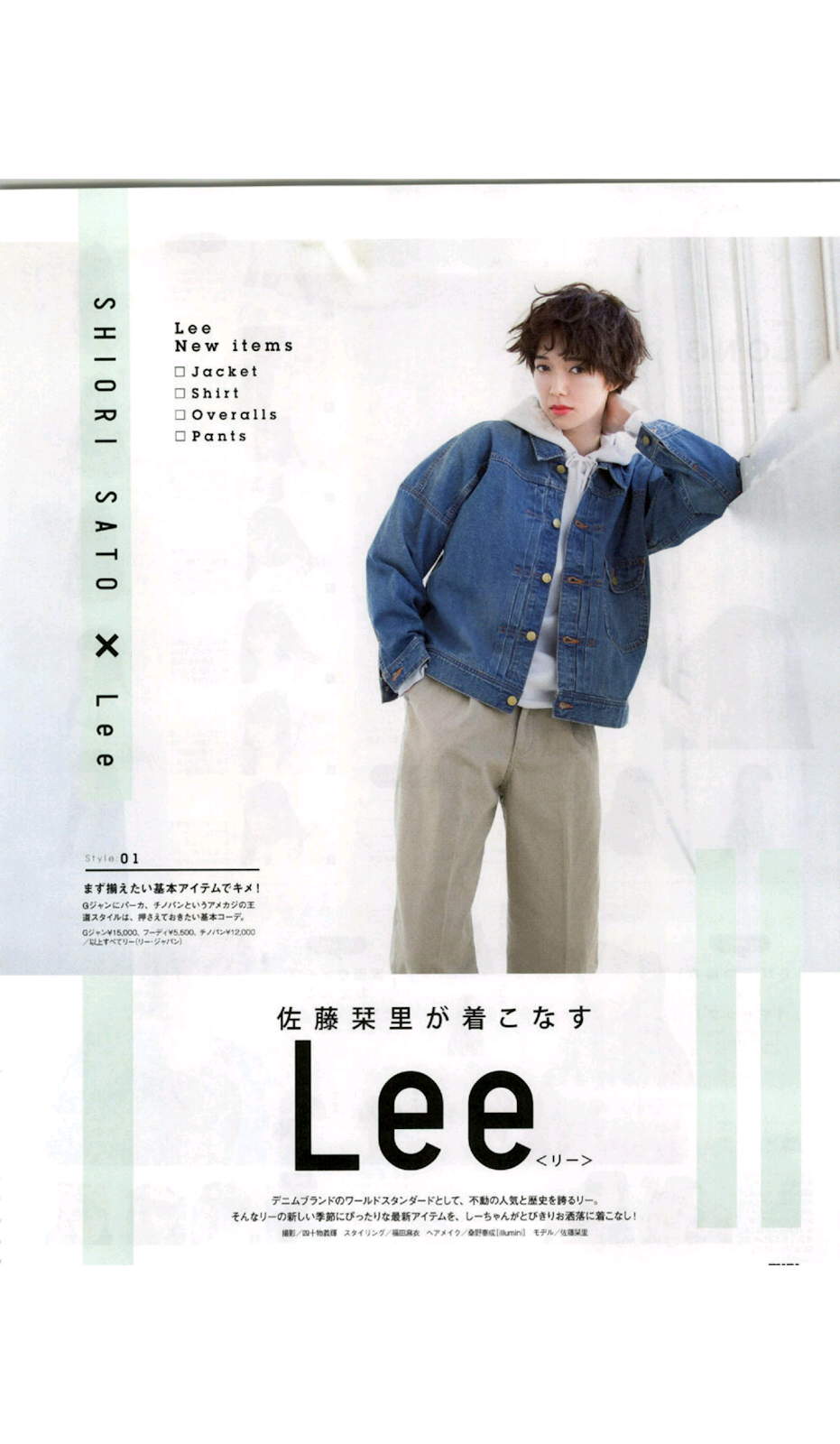The advertisement for the Lee brand features a female model with short brown hair and red lipstick, standing slightly off-center to the right against a white wall. She's wearing an unbuttoned blue denim jacket with a white hooded top underneath, and khaki pants. The background is a mostly white marbled texture. 

The left side of the image includes notable text elements: at the top left corner, "Lee New Items" in small text with an unchecked list of items (jacket, shirt, overalls, pants). To its left, running vertically in black text, it reads "Shiori Sato X Lee," indicating a collaboration. In the bottom left corner, there is additional text that's too small to decipher. The overall layout emphasizes the branding and collaborative nature of this fashion advertisement.